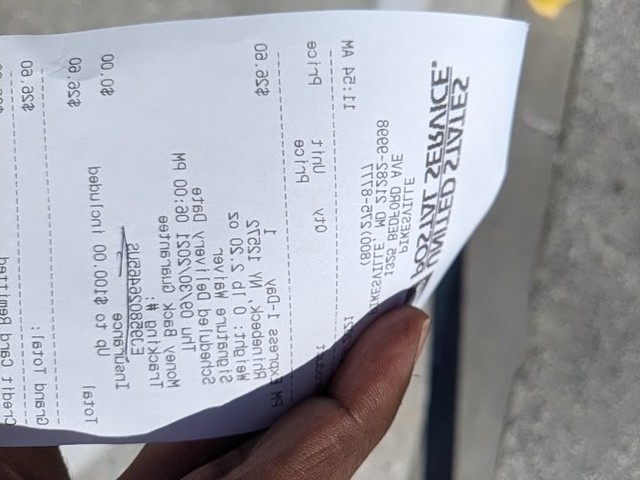This color photograph showcases a close-up view of an African American person holding a United States Postal Service receipt between their index and middle fingers, with the index finger prominently visible on both sides. The bright lighting reveals the text on the receipt in a mirror image, making everything appear backwards. Key elements such as "Pikesville, Missouri" and "Bedford Avenue" can be discerned, along with some financial details including a cost of $26, possibly for express mail, and other monetary values like "06.62" and "00.001" dollars. The receipt, held sideways in the frame, includes features like a money-back guarantee and an 800 number, and appears to have a date of May 24, 2011. The background is a concrete gray, suggestive of a wall, with a small, indistinguishable yellow mark at the top right corner.